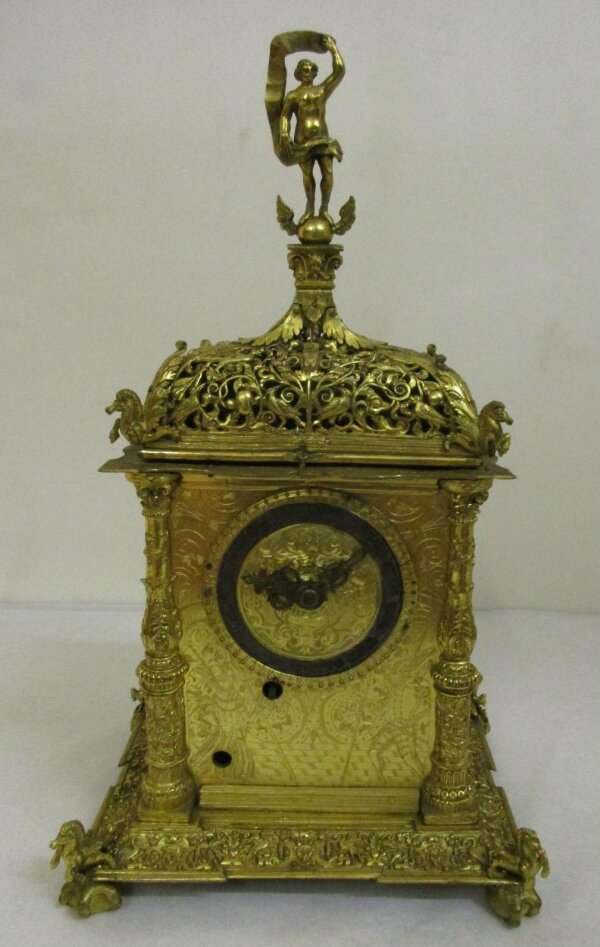The image showcases an ornate antique clock made primarily from a gold-toned metal, possibly brass. The clock stands out against an off-white background and depicts intricate designs filled with floral and foliage motifs. It has a sturdy square base with detailed engravings, and little legs at the front. The central body of the clock is adorned with elaborate scrollwork patterns, framing a black circular clock face with a gold center and black hands pointing to around ten past nine. Midway up the clock, two golden columns flank the main structure, providing a balanced symmetry.

At each upper corner of the clock are decorative elements resembling horse heads or partial horse bodies, adding to its unique charm. The pinnacle of the clock features an elaborate decoration resembling a crown, surmounted by a person standing on a winged ball. This figure appears to be holding a draped banner or piece of material over their head, giving the impression of dynamic motion. The detail and craftsmanship in the figure’s design, combined with the ornate filigree work and textured patterns throughout the piece, accentuate its antique and luxurious aesthetic.